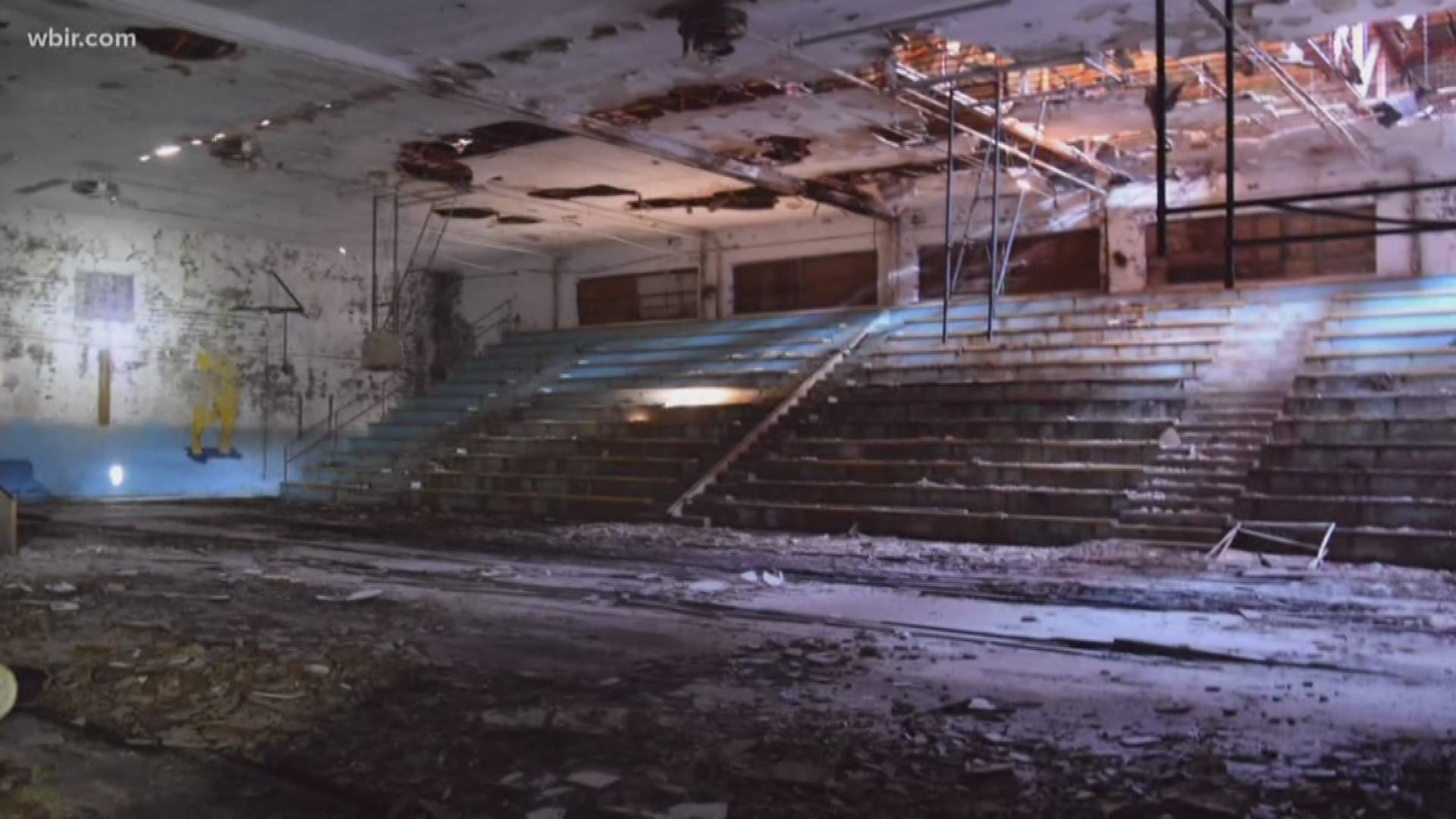This photograph, likely screenshotted from a video on wbir.com, captures a dark, abandoned gymnasium in severe decay, possibly an old high school gym. The once vibrant stadium bleachers are now heavily discolored and coated with debris, including gravel and pieces of the rotted ceiling. The ground, a chipped and worn concrete surface, is littered with ceiling remnants. Numerous holes punctuate the roof, exposing support structures and rusted areas, giving the impression that the entire ceiling could collapse at any moment. The left wall, with its faded paint and peeling areas, stands decorated with a lone remaining basketball hoop and a faded blue section, possibly featuring a painting of a person in yellow. The whole setting suffers significant water damage and decay, reflecting years of neglect and abandonment.